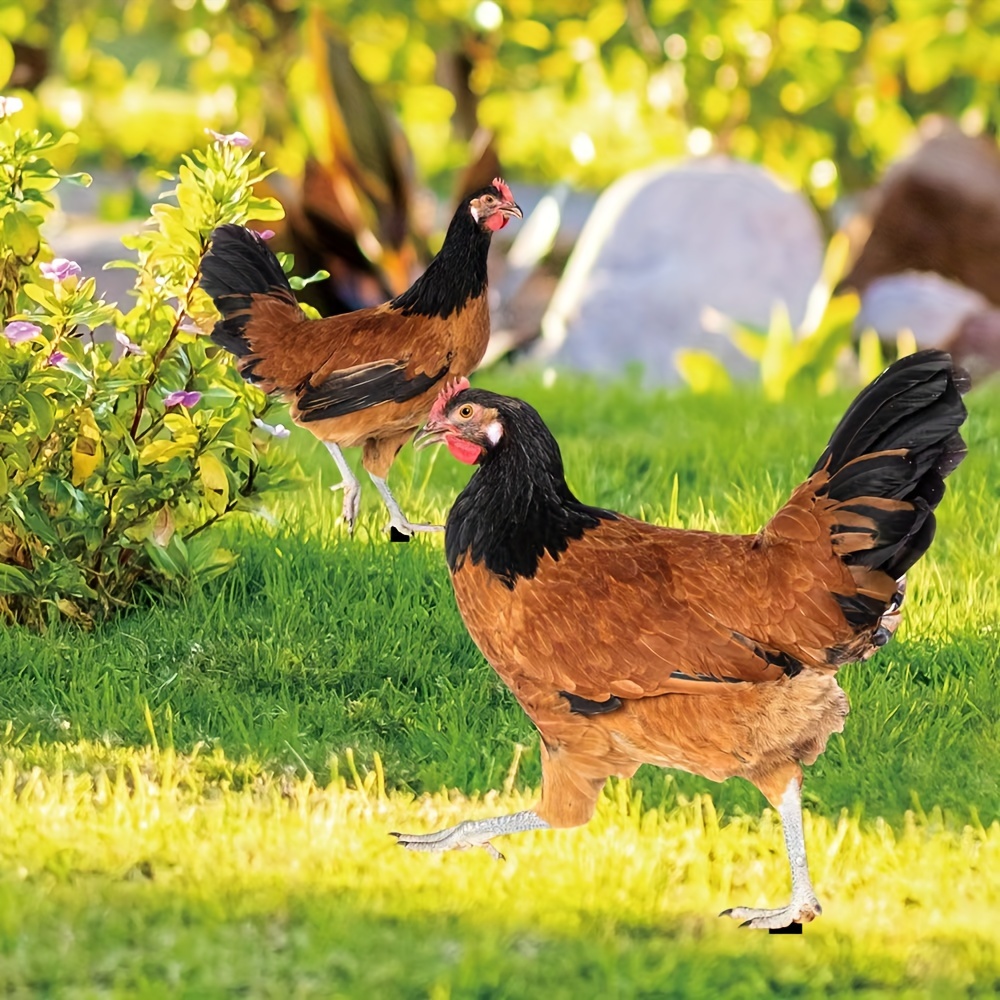In this daytime outdoor scene, the image features two roosters grazing in what appears to be a garden or backyard with farm-like elements. The vibrant sunlight illuminates the area, highlighting the grassy foreground, which transitions from a bright yellowish-green closest to the camera to a more vivid green farther back. On the left side, a small bush adorned with delicate pink flowers adds a splash of color.

In the foreground at the bottom right, one rooster, with a striking combination of black feathers on its head and tail and brown feathers on its body, stands out prominently. It has a red mohawk-like crest on its head and distinctive white legs, with its right leg forward and left leg on the grass. The sunlight casts a bright sheen on the grass where it stands.

In the middle left background, another rooster with similar brown and black feather patterns faces the right. This rooster also has red markings around its face and a black tail, and its feet and legs bear a somewhat animated appearance with a grayish tint and black talons. Nearby, to the rooster's left, a green and yellowish plant stretches upward and slightly to the right.

The far background of the image is blurry, but you can discern a mix of green and yellow hues, along with indistinct shapes, including a notable white rounded object on the far right and larger stones in white and brown tones. The overall scene captures a tranquil moment in a sunlit, lively backyard setting.